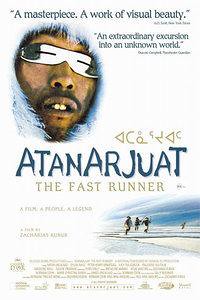This detailed movie poster for "Atanarjuat: The Fast Runner" features a striking white background with an abundance of text. Dominating the top left corner is the face of an indigenous man, framed by the fur hood of his coat. His silver glasses have lenses that are just tiny slits. Below this, in the center, the movie title stands out in large blue font, spelling "A-T-A-N-A-R-J-U-A-T." Beneath the title, in lighter brown font, the subtitle reads "The Fast Runner." Scattered around the poster are critical accolades, including quotes such as "A masterpiece, a work of visual beauty," and "An extraordinary excursion into an unknown world." The bottom right of the poster depicts several people sprinting across an icy landscape. Additional text and small logos near the bottom detail the film's credits, although they are largely illegible. The overall composition suggests a powerful and visually stunning narrative set in a wintery expanse.